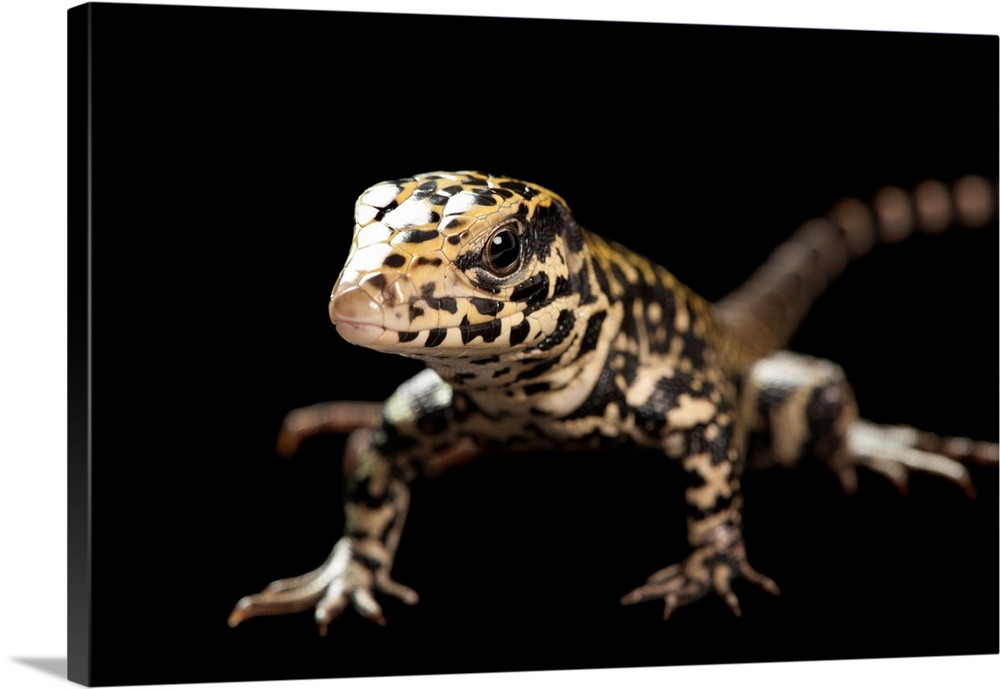This is a detailed photograph printed on a canvas, evident from a visible side edge hinting at its 3D nature. Set against a stark black background, the central subject is a lizard with vivid yellow scales and contrasting black dots. The lizard is oriented forward, slightly turned to the left, with its head sharply in focus while the rest of its body, particularly the tail, fades into a blur. Notably, its tail exhibits distinctive black ring patterns. The claws on both its front and back feet are clearly visible, with five on each. The speckling on the lizard's body starts finer near the head and appears larger towards its legs. The image highlights the lizard's detailed texture and coloration, rendering it a striking and lifelike depiction.